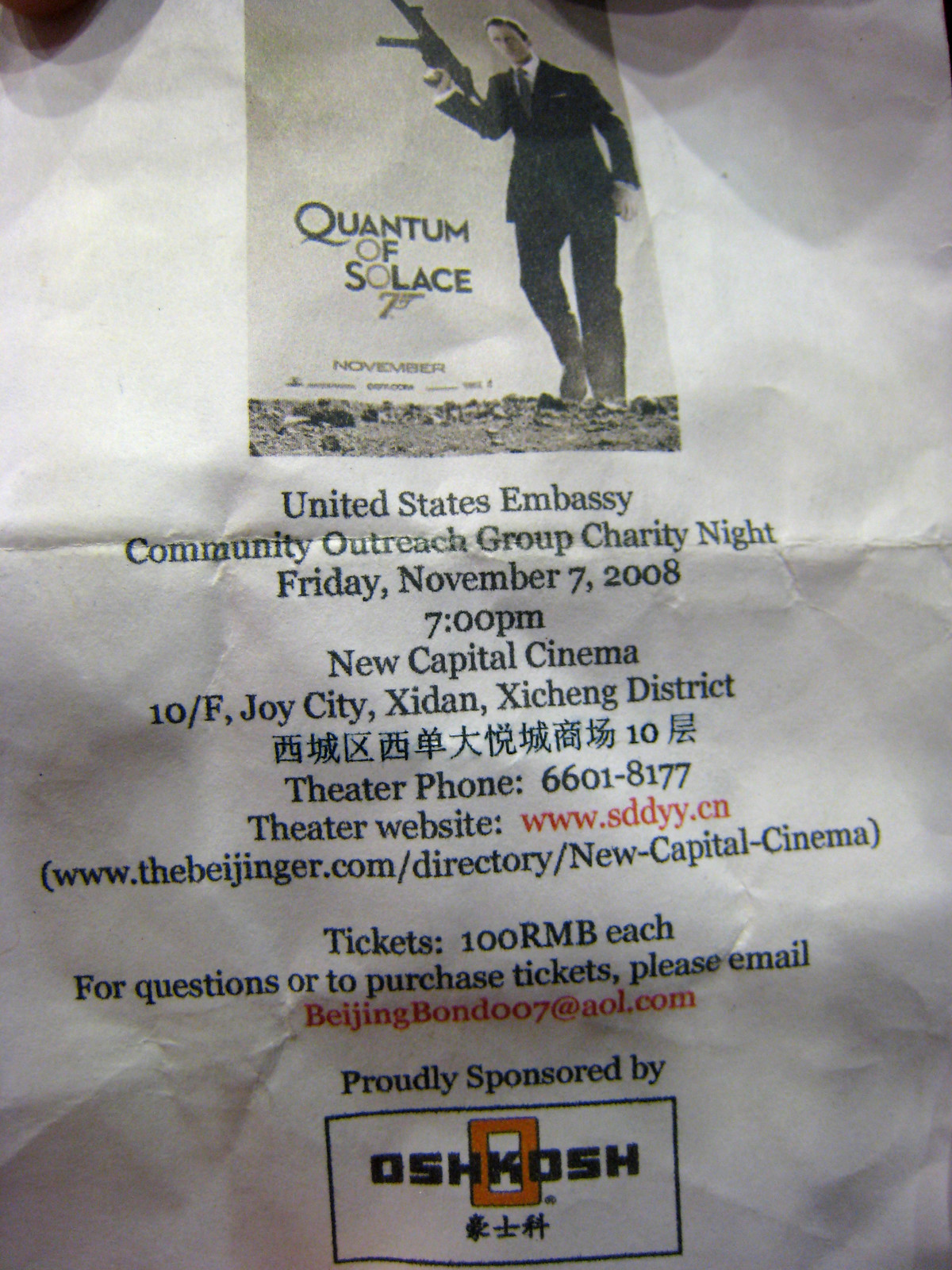A crumpled flyer for a United States Embassy Community Outreach Group Charity Night, showcasing a screening of the James Bond movie "Quantum of Solace," held on Friday, November 7, 2008, at 7 p.m. at the New Capital Cinema, 10th Floor, Joy City, Zhejiang District in China. The gray and white poster features a small image at the top of Daniel Craig as James Bond, wearing a suit and holding a machine gun while standing on rocky terrain. Below the image, the flyer contains black text detailing event information, including a theater phone number (6601-8177), theater website (www.sddyy.cn), and additional contact and ticket purchase details (tickets at 100 RMB each, email: BeijingBond007@aol.com). The flyer also includes the website www.thebeijinger.com/directory/New Capital Cinemas and is proudly sponsored by Oshkosh.